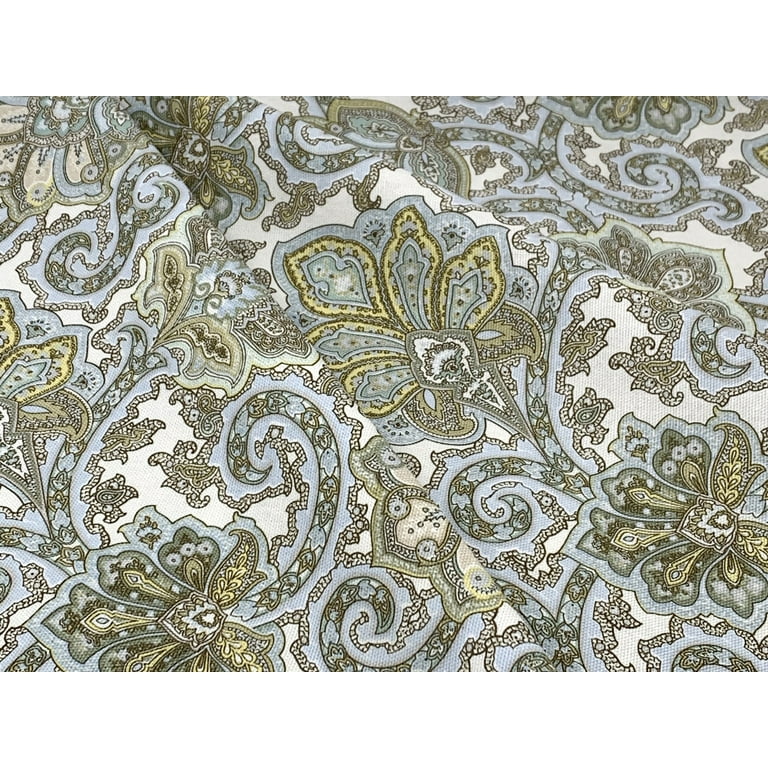This photograph showcases a white fabric, potentially a bed sheet or tablecloth, adorned with intricate and non-repeating floral patterns. The design features large flowers, stems, and leaves, with colors including blue on the outer part of the petals, brownish hues inside, and touches of green and bluish-gray. Additionally, there are purplish and yellowish-green shades throughout the fabric. The fabric is slightly crinkled and folded, adding a textured dimension to the image. Dominating the center is a distinctive motif, resembling a diamond or downward-pointing triangle, framed by five leaves—four from each side and one larger leaf at the top—enhancing its intricate and complex design.